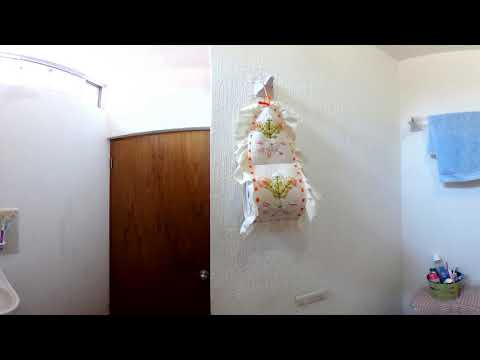The image depicts a bathroom with predominantly white walls that feature subtle variations in texture. The left wall is smooth white, while the right wall reveals faint streaks of underlying wood grain. Mounted on the right wall is a white holder from which hangs a decorative pink and white bag, adorned with delicate red dots and featuring two embroidered trees with pink blossoms. Centrally positioned in the room is a vertical brown wooden door with a silver handle, adding a touch of warmth to the space. To the left of the door, the edge of a white porcelain sink is visible, with what appears to be a piece of artwork above it, distinguished by its pink and purple hues. On the right side of the room, a toilet is present, topped with a green basket storing various toiletries. Above the toilet, a towel rack holds a baby blue towel, adding a calming color contrast. A knitted decoration enhances the room’s cozy ambiance, making it a welcoming space.